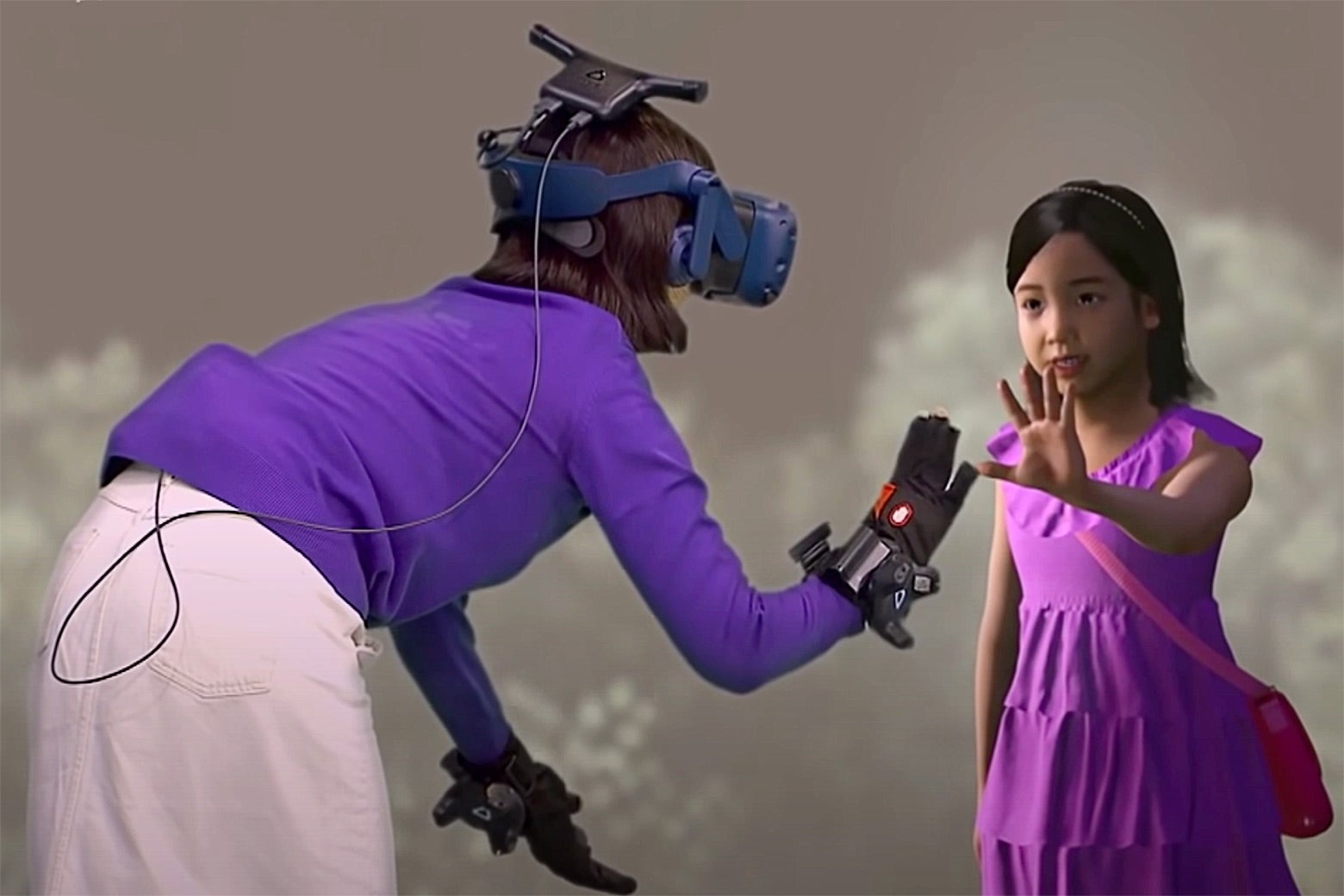The rectangular image, approximately six inches wide and three inches high, depicts a woman and a young girl against a light brown backdrop with a purplish undertone, and vague white bush-like shapes on either side. The woman, positioned with her back towards us, is bending forward at the waist, wearing a long-sleeved purple top and a white skirt. She dons a cumbersome virtual reality headset connected by a wire to a pack at her back, and gloves with metal designs around her wrists. The young girl, facing the woman, appears as though she is part of a simulation. She is Asian, with short black hair, purple eyes, and a sleeveless purple dress, accessorized by a cross-body pink handbag. Both their hands are extended towards each other, creating a touching connection. The background behind them transitions into a cloudy, light brown sky, enhancing the otherworldly atmosphere of the scene.